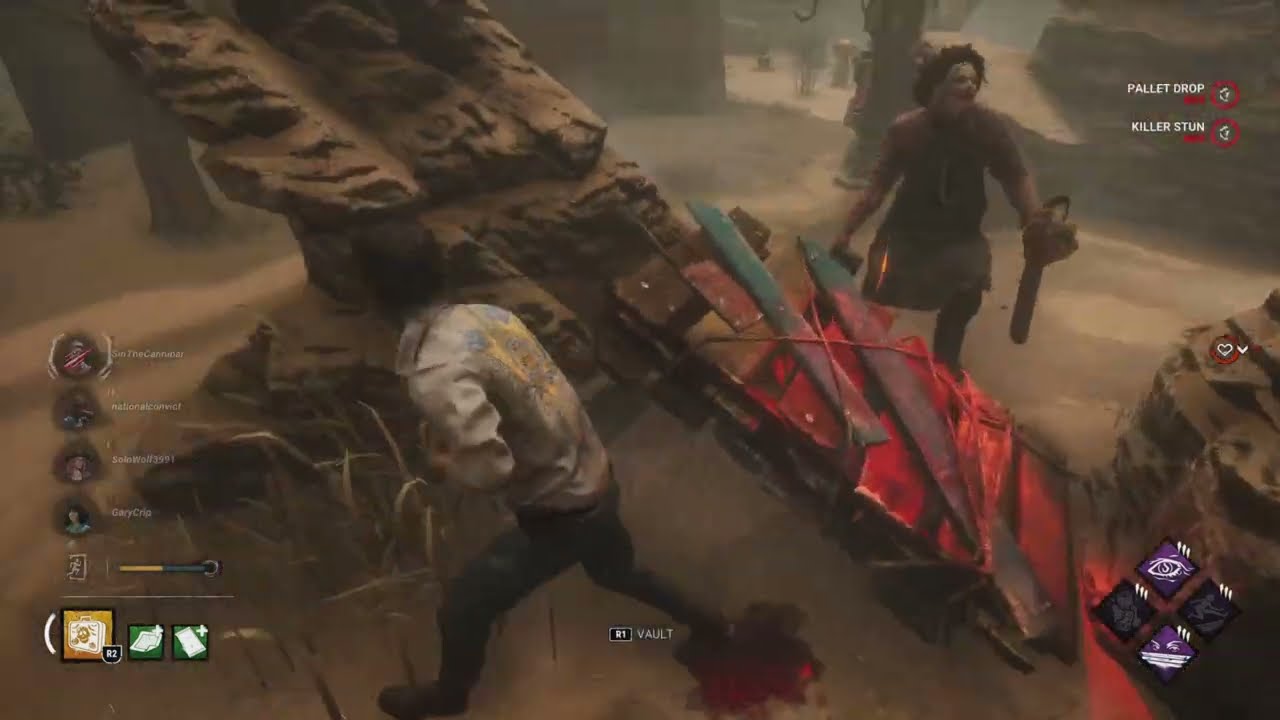The image is a horizontal rectangular screenshot from a gory video game. The background is dominated by a large rocky structure extending from the upper left, with wooden boards smeared with red blood and bits of steel. To the right, a tall, creepy figure with black hair, wearing a butcher’s apron and a mask, holds a chainsaw in his left hand. This menacing figure appears to be one of those classic horror characters, reminiscent of Jason. In the middle to the left side, the main character, dressed in a dirty white shirt and jeans, is running away towards the left, showing visible bleeding from his right leg, which just stepped on a bloody patch on the ground. The scene is set around some trees or a concrete structure, further adding to the eerie ambiance. A wooden pallet is leaned at an angle between two rocky pillars, separating the two characters. There's a heads-up display (HUD) including four triangular icons at the bottom right, as well as other gameplay elements like a few purple icons at the bottom right and inventory icons on the bottom left. The top right features white text with the words “Pallet Drop” and “Killer Stun,” enhancing the immersive gameplay experience.